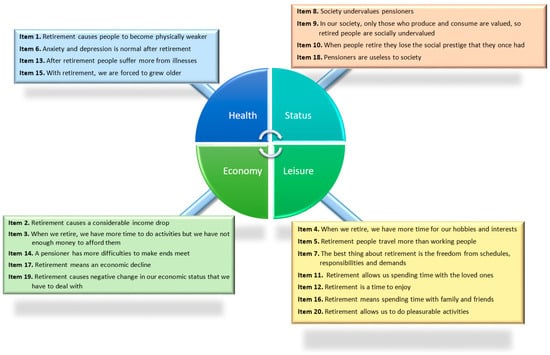This educational graphic features a central circle divided into four segments: Health (blue), Status (teal), Economy (light green), and Leisure (green). Each segment’s lines extend outward to four rectangles, each packed with detailed textual information. Items listed in these boxes include statistical insights and observations, such as "retirement causes people to become physically weaker" under Health, and "society undervalues pensioners" under Status. The colorful segments and connecting boxes create a visually engaging way to explore complex societal and economic topics, ideal for educational purposes.